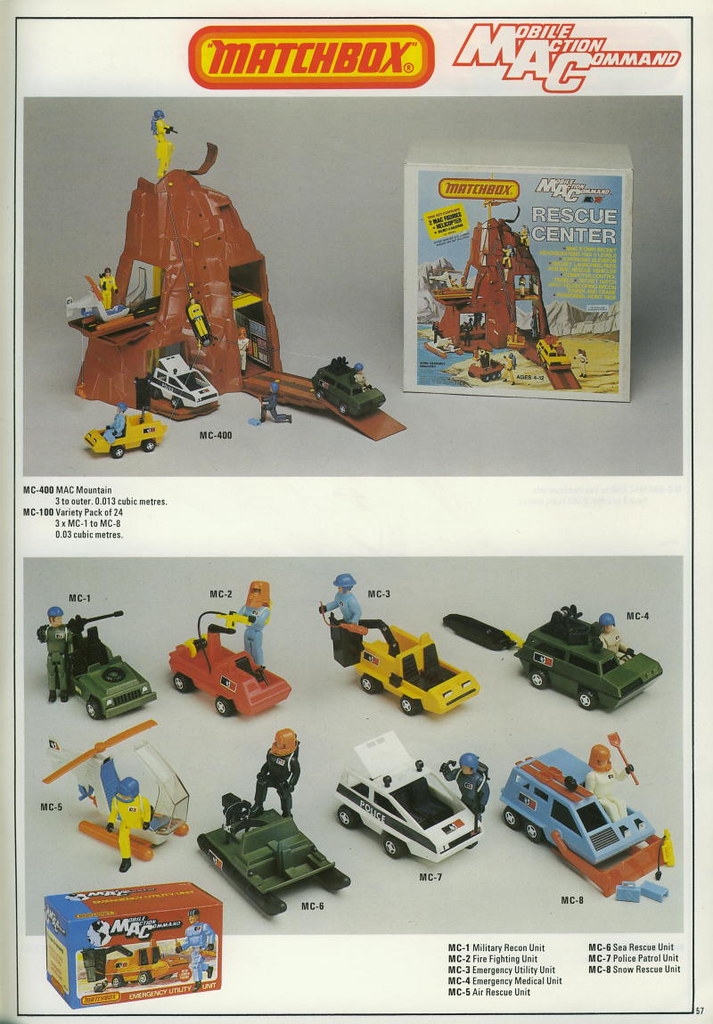The image is an advertisement for Matchbox's Mobile Action Command (MAC) Rescue Center. At the top, the ad features the iconic Matchbox logo—a red rounded rectangle with an orange rounded rectangle inside, filled in yellow and containing the word "Matchbox." It prominently displays the MAC Mountain, a brown mountainous structure from which various rescue vehicles are emerging, showcasing their functionality once fully assembled. These vehicles include a green tank, a white vehicle, a helicopter, and several others, each paired with an action figure. The set includes different units such as Rescue, Police Patrol, Snow Rescue, Air Rescue, Emergency Medical, and Firefighting. The ad contains detailed descriptions and a legend that identifies specific vehicles like the Military Recon Unit and corresponding features. Alongside the toy photos, there is the packaging that highlights the MAC theme and various unit names, reinforcing the playset's comprehensive rescue capabilities. 

Overall, the advertisement combines visual appeal with detailed information, emphasizing the multifunctional aspect of the Matchbox Rescue Center, where various rescue operations are vividly brought to life.